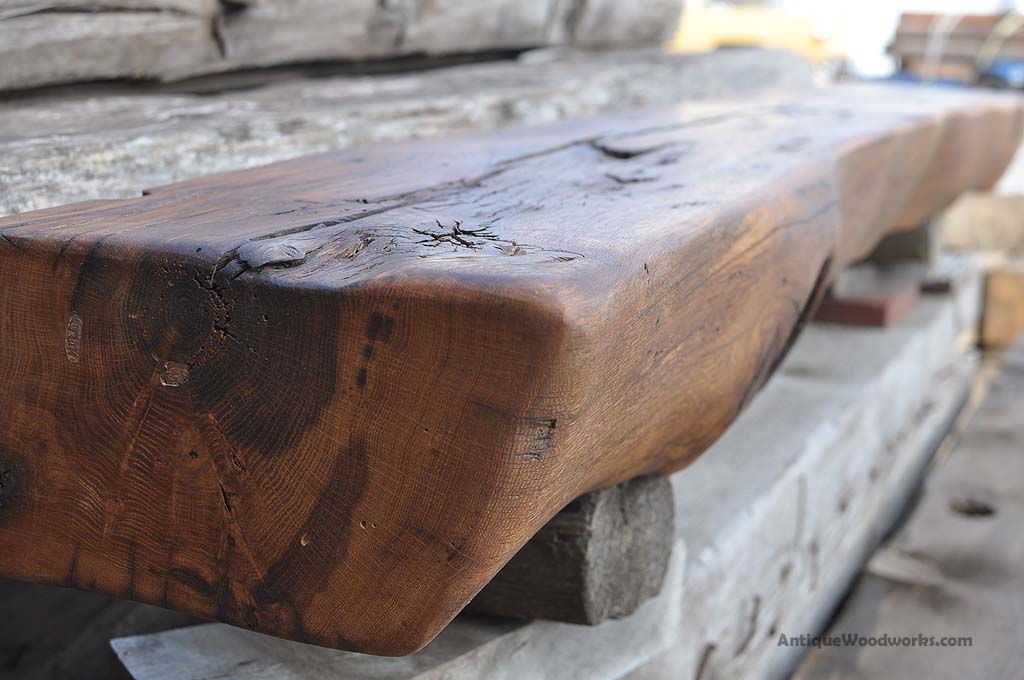In this outdoor photograph, a close-up shot captures a rustic, handcrafted wooden bench, seemingly carved from a large, single piece of medium-grain wood, possibly a stump. The wood exhibits rich, dark brown tones with natural grain patterns and several dark cracks, adding to its antique appeal. This bench sits atop a layered base comprised of a darker wooden piece and white concrete, which displays visible black cracks. To the bottom right of the bench, black lettering reads "AntiqueWoodWorks.com." The bench is positioned diagonally across the image, stretching from the bottom left to the top right, while the background features blurry elements such as brown shelving and a machine. The scene suggests a workshop or outdoor patio setting, hinting at the craftsmanship that went into creating this antique wooden piece.